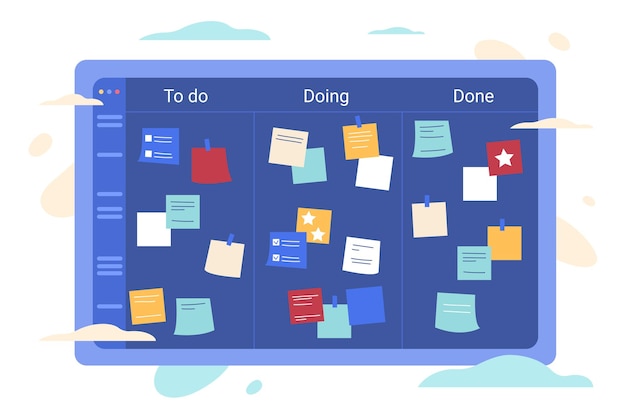This image showcases a computer-generated, cartoon-like to-do board with a rectangular purple background and three clearly defined columns: "To Do," "Doing," and "Done." Each column is separated by lines, organizing an array of colorful sticky notes. 

The "To Do" column on the left features several sticky notes in colors including blue, light blue, red, white, yellow, and orange, all marked with lines that suggest writing. The "Doing" column in the center consists of approximately 12 sticky notes in a similar variety of colors — orange, blue, light blue, red, and yellow — and some include check marks and stars. These notes represent tasks currently in progress.

On the right side is the "Done" column, where completed tasks are displayed on sticky notes. Notably, one red note features a prominent white star. In total, there are seven notes in "To Do," ten in "Doing," and eight in "Done." The background is filled with whimsical cloud-like shapes in blue-green and beige hues, adding to the overall cartoon aesthetic of the image.